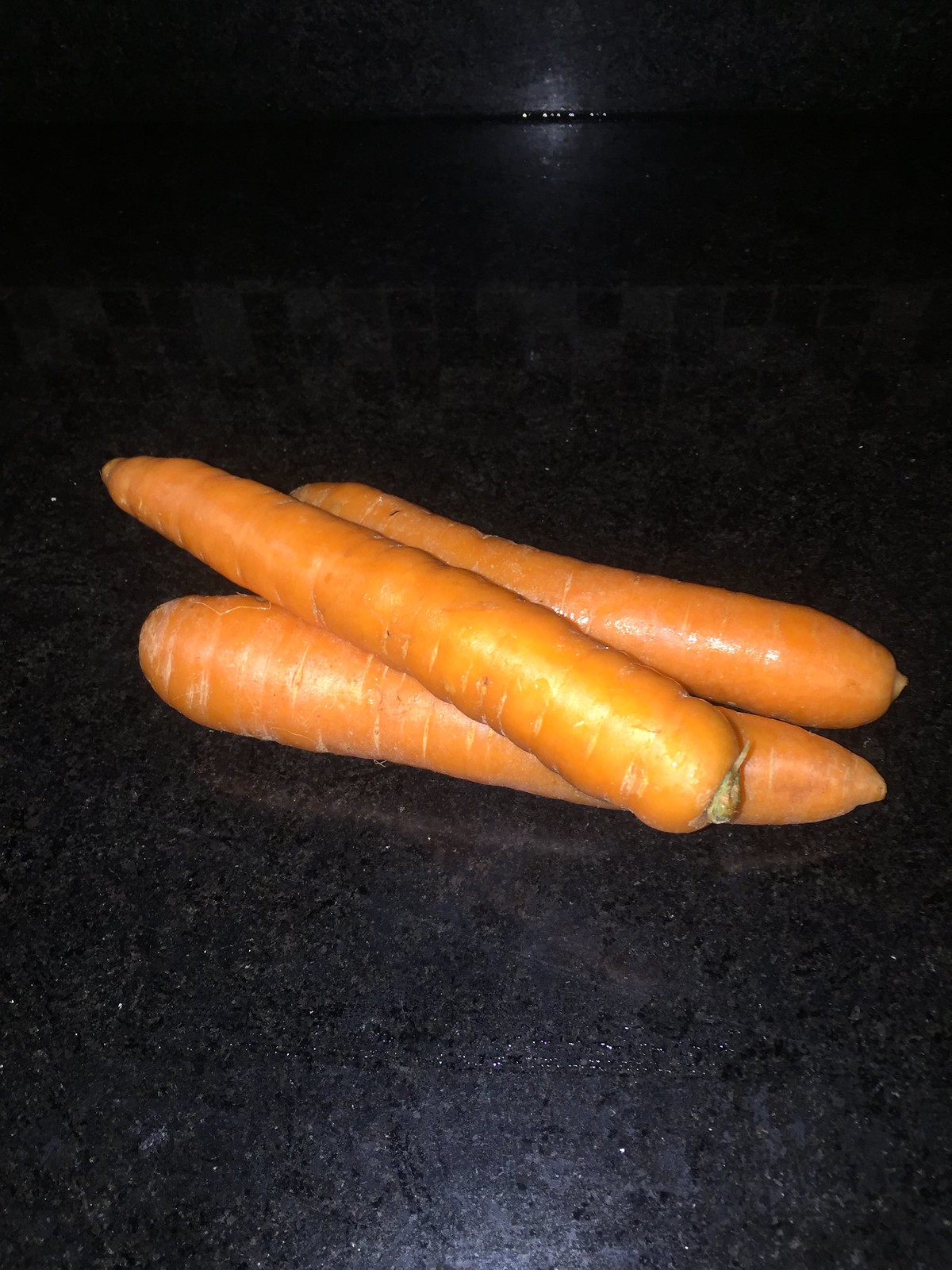This close-up color photograph features three vibrant orange carrots on a shiny black granite countertop, set against a dark background. The carrots are arranged horizontally in a slightly diagonal manner, with two lying side by side and the third one placed on top, crossing from left to right. Despite having their stems removed, small green nubs are still visible. The clean, slightly imperfect carrots, possibly just washed after being pulled from the ground, reflect the light strongly—one even reflecting a yellowish tinge. The background includes tiny illuminated lights at the top and a faint glare at the bottom, possibly from a flash, with hints of a checkerboard pattern visible from reflections. The countertop shows some dust and minor scratches, further highlighting the pristine state of the carrots.